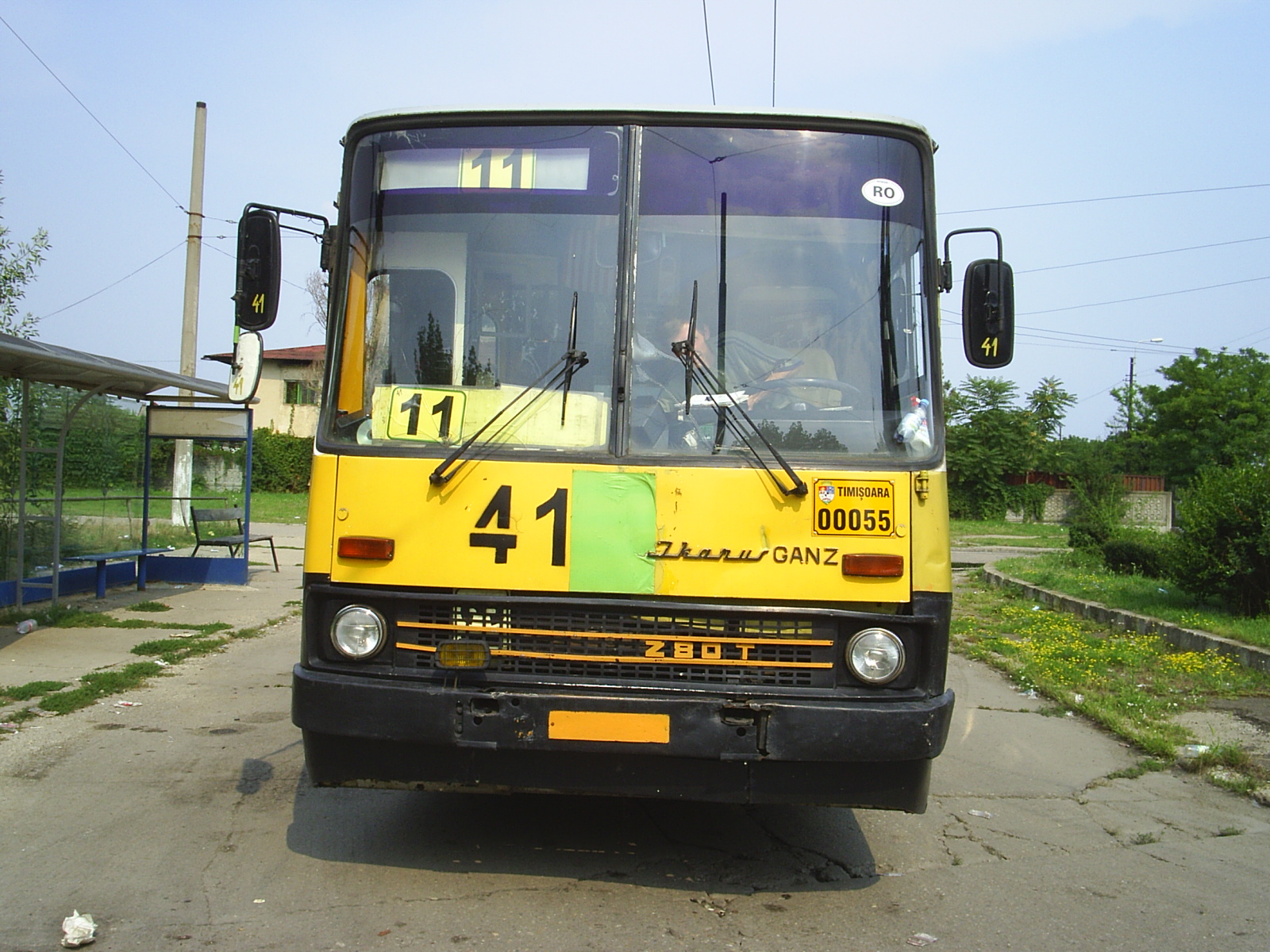The photograph captures a vibrant daytime scene featuring a commuter bus on a cracked and weathered concrete road. The horizontal rectangular image showcases a bright blue sky with sparse white clouds overhead. The bus, prominently positioned at the center, faces the camera and fills much of the upper frame space. This yellow bus, accented with a black bumper, visibly displays a split windshield with black frames and central divider, topped with black windshield wipers. The front of the bus features two large, transparent windows framed in black, and both windows and the bus's front itself are rich with detail: the left window displays a small yellow sign with the black number 11, while a gray bar with white centrally located and marked with the same number anchors the top left corner.

Below the windows, the front panel of the bus shows the number 41 in black text, flanked by orange lights at the lower corners. The black grill beneath the yellow panel features the text "Z bot" in orange, framed by two additional lights. The road beneath the bus is broken and worn out, sprouting patches of grass.

The surroundings offer a mix of urban and natural touches: to the left stands a blue bus stop with a bench and a shelter, with a telephone pole and power lines stretching skyward nearby. On the right, colorful flowers emerge from cracks in the concrete near a small barrier, transitioning into a grassy area backed by a row of trees and scattered bushes. The far end of the scene reveals a yellow house with red roof partially obscured by vegetation, adding to the idyllic yet bustling composition of the setting.